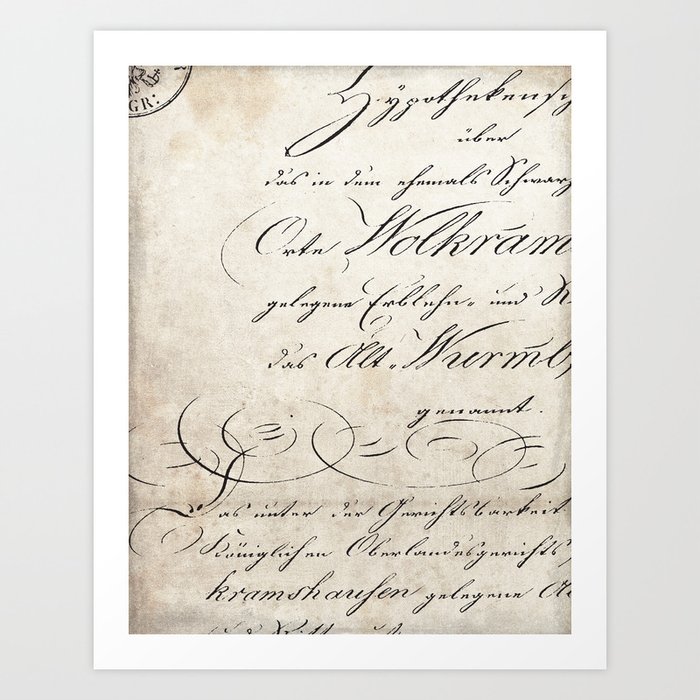The image features an artful display of calligraphy on a discolored, coffee-stained piece of paper. This old and textured paper is framed by a thick, white border approximately 2 to 3 inches wide, which is superimposed on a gray background. In the top left corner of the paper, there is a semicircle with the letters "GR," resembling a stamp or seal, though this mark is partially cut off. The main body of the page is dominated by elegant yet unreadable calligraphy in a cursive-like script, making it difficult to discern the language or specific words. About three lines down, the word "WOLKRIM" stands out amidst the ornate writing. The writing follows a right-aligned format, running from the top to the bottom of the page. In the lower middle section, there are incomplete calligraphic circles, and beneath them, more detailed and tightly lined writing that is slanted to the right.